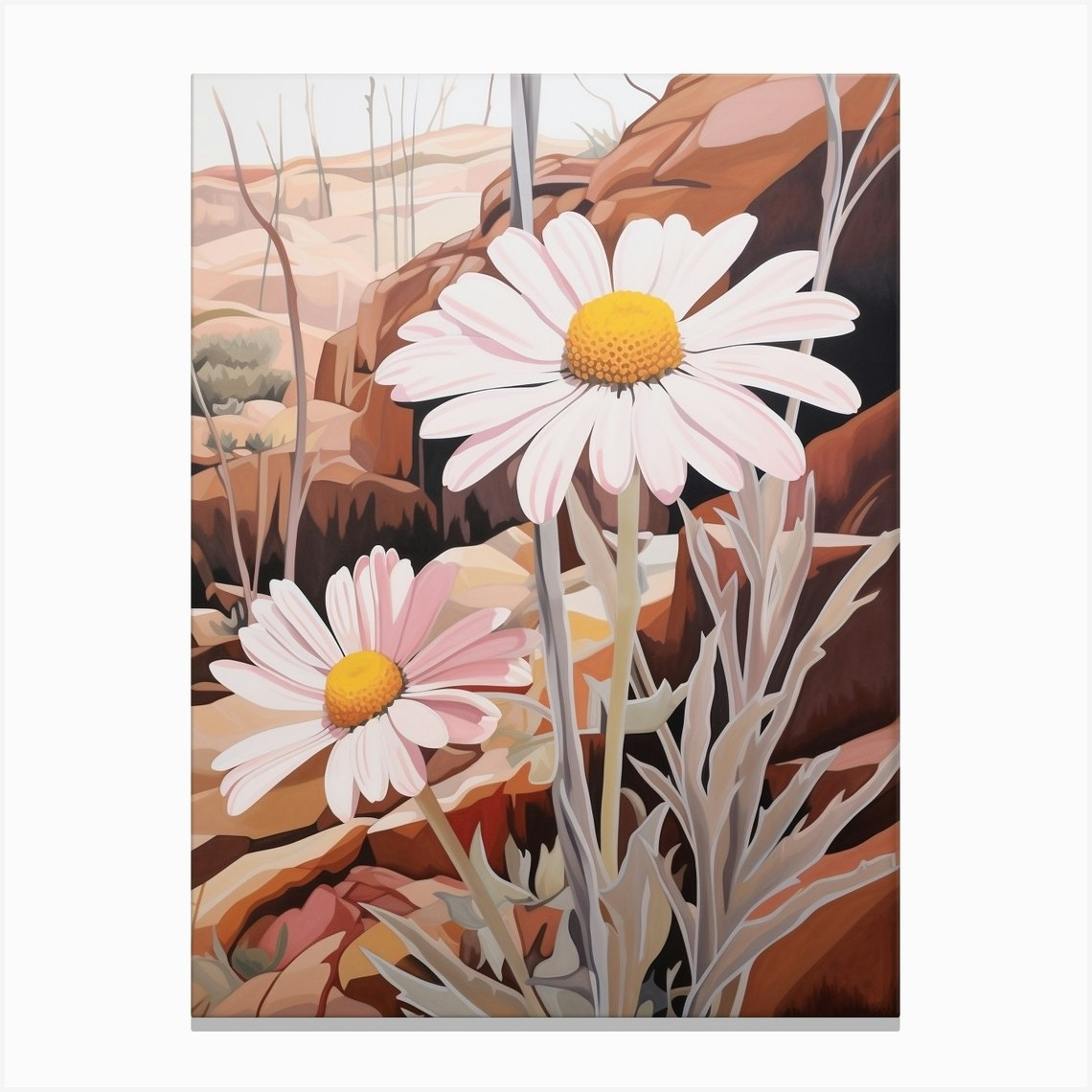The image appears to be a detailed watercolor painting depicting a pair of daisies set against a rocky, desert-like background. The focal point is on two white daisies with numerous petals extending from a vibrant yellow center, one standing taller than the other. The shorter daisy exhibits a subtle pink hue on some of its leaves, likely due to the shadow cast by the taller flower. The stems and leaves are rendered in muted, nearly khaki or army green shades. The background features a variety of light and dark brown rocks, enhancing the arid, rugged feel of the landscape. Distant rocky formations add depth to the composition, while a light sky completes the scene. Sparse vegetation, including dried branches or trees and low bushes, are scattered throughout, contributing to the painting's natural, desolate ambiance.